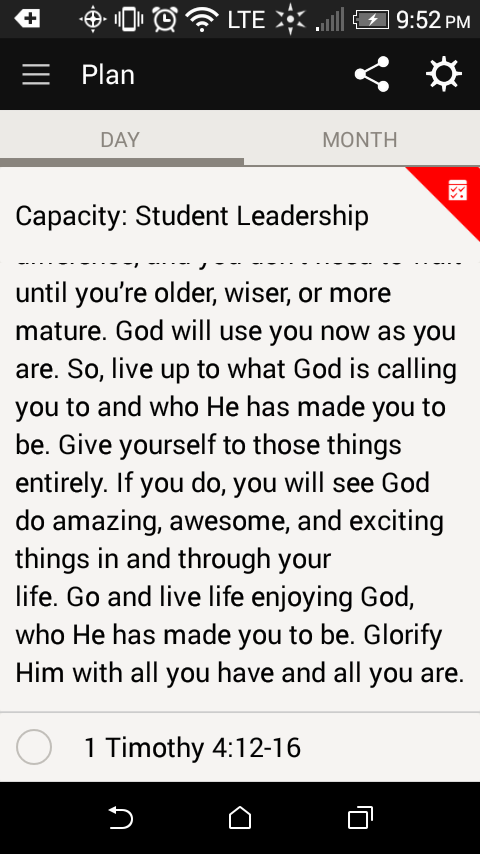The image is a multi-color screen grab taken from a phone displaying a Bible verse aimed at student leadership. At the top of the image, a black banner shows various phone indicators, such as the time (9:52 p.m.), battery level, phone signal with one bar, LTE status, full internet connection, and icons for alarm and vibrate modes. The middle section contains the primary content, a passage with black text that begins with “capacity student leadership” and instructs the reader: "Until you're older, wiser, or more mature, God will use you as you are. So live up to what God is calling you to and who he has made you to be. Give yourself to those things entirely. If you do, you will see God do amazing, awesome, and exciting things in and through your life. Go and live life enjoying God who has made you to be. Glorify him with all you have and all you are." The passage is cited as 1 Timothy 4:12-16. The bottom of the screen also shows a black navigation banner with icons, including a left-pointing curved arrow, a pentagon shape, and two stacked squares. The image contains a mix of colors, primarily shades of black, white, red, and some tan elements, and gives the appearance of a screenshot from a notes app concerning student leadership and Christian faith.